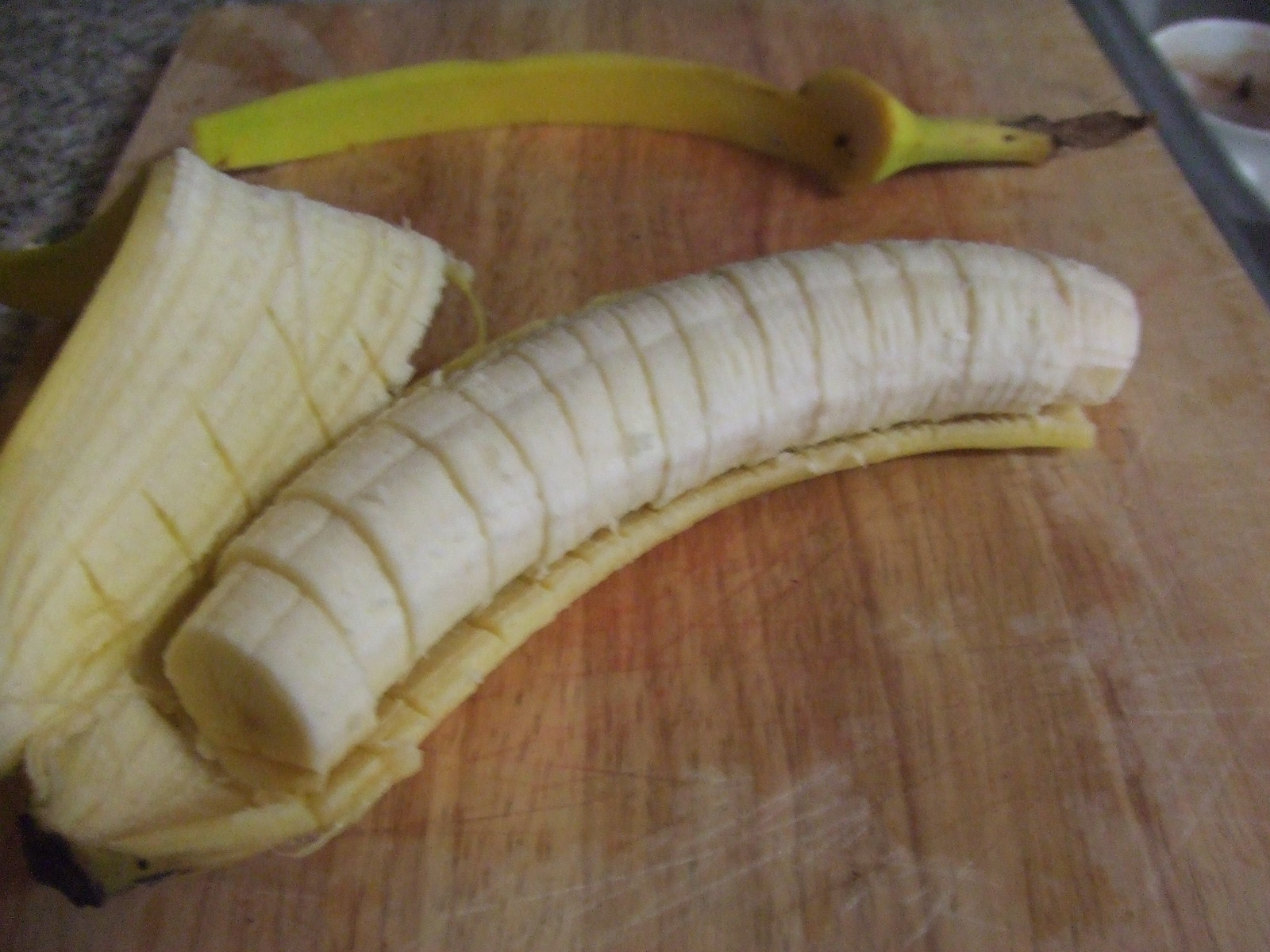The image depicts a person in the process of slicing a banana on a wooden cutting board. The banana, partially peeled, lies diagonally across the center of the image, stretching from the bottom left to the middle right. The peel is separated and splayed out, extending from the bottom left to both the middle and top right. A knife suggests recent activity, with several neatly cut banana slices scattered on the board. The cutting board is placed on a kitchen countertop, visible on the left side of the image, and the edge of the floor, which appears to be wooden, can be seen. On the right side of the image, there is a white cup or candle, adding a touch of homeliness to the scene.